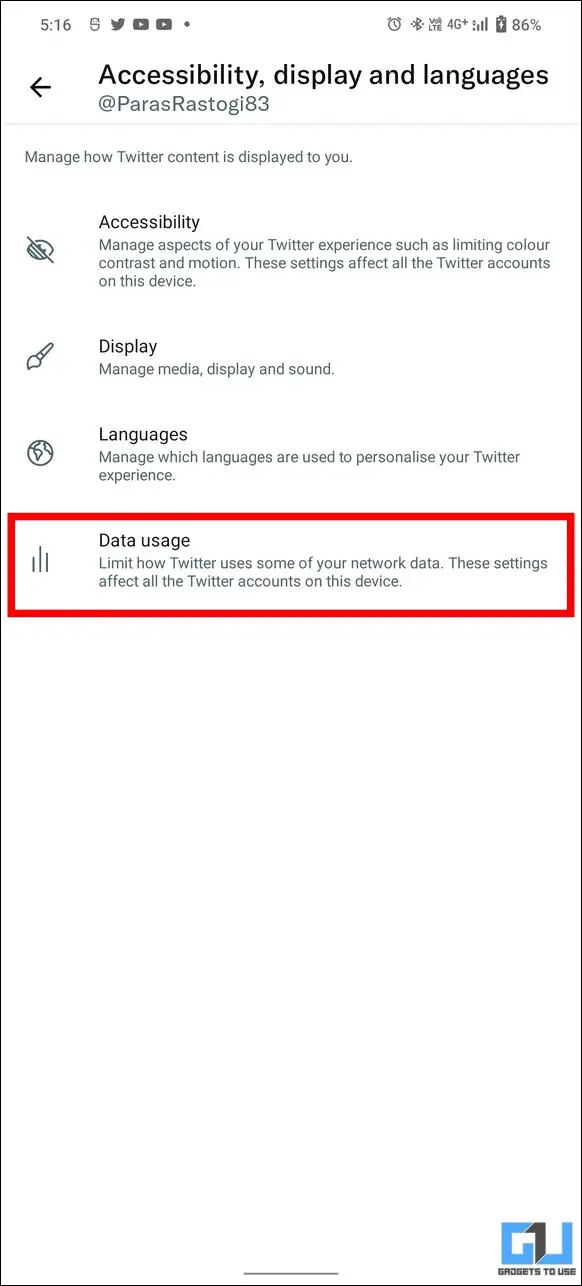This image is a screenshot taken from a cell phone displaying the settings menu of the Twitter app. The time at the top center reads 5:16, with various icons for social media and a battery life indicator showing 86% in the upper right corner. Below this, a navigation instruction reads "Accessibility, Display, and Languages" with a right-pointing arrowhead.

The next line shows "@ParasRostico GI 83" in small text. Beneath a faint gray dividing line, there's a description reading "Manage how Twitter content is displayed to you," followed by four selection options: Accessibility, Display, Languages, and Data Usage.

The "Data Usage" option is highlighted with a red rectangle, emphasizing the description: "Limit how Twitter uses some of your network data. These settings affect all the Twitter accounts on this device." In the bottom right corner of the image, a blue and gray emblem features the stylized text "Gadgets to Use," with a distinctive logo incorporating the letters G, T, and U.